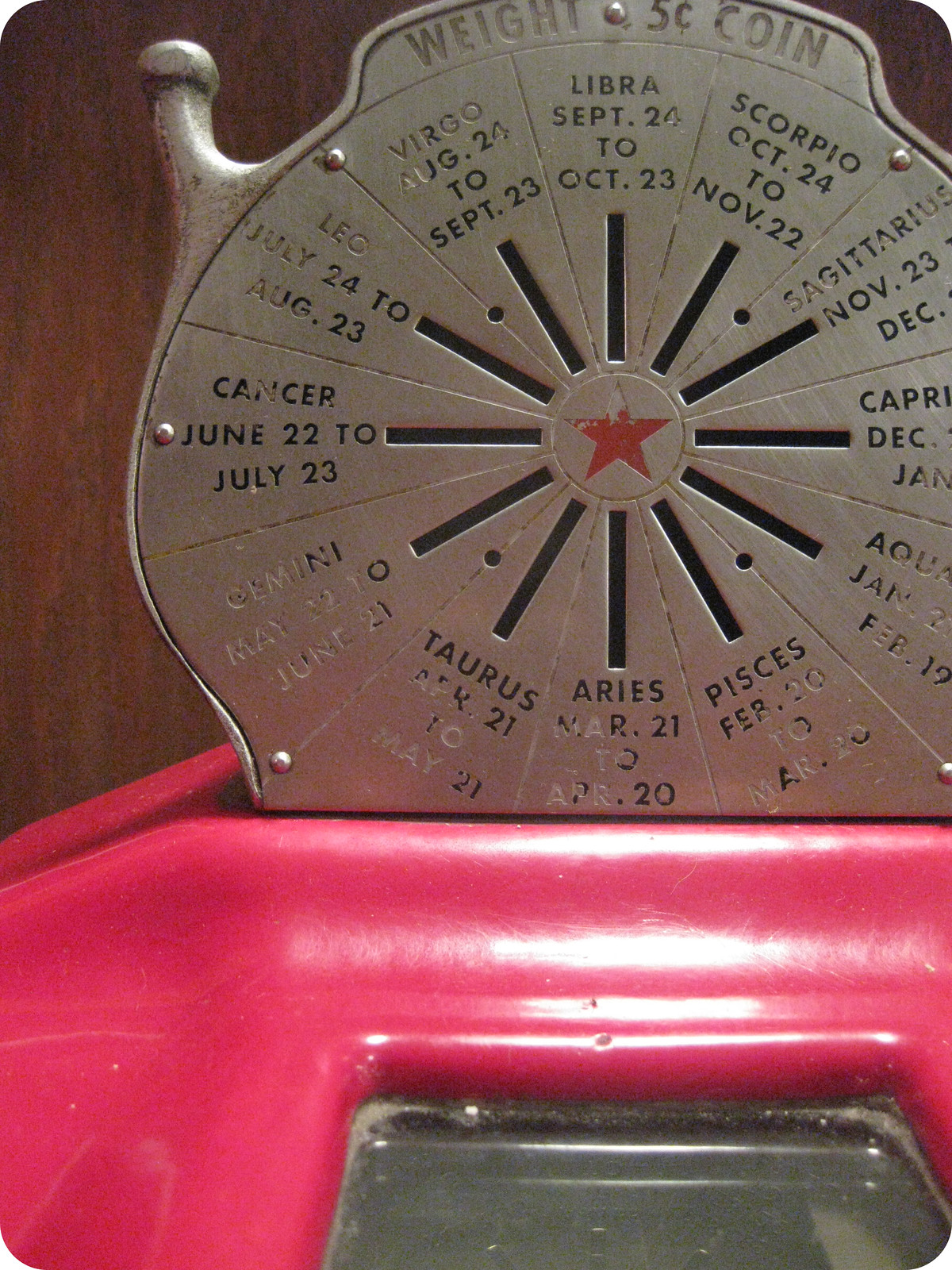This is a close-up photo of a vintage horoscope weight machine. The base of the machine is red, and above it, there's a large round metal plate with 12 slots, each labeled with a zodiac sign and the corresponding date ranges. Starting from the top and going clockwise, the zodiac signs and dates include Libra (September 24th to October 23rd), Scorpio (October 24th to November 22nd), Sagittarius (November 23rd to December 21st), Capricorn (December 22nd to January 20th), Aquarius (January 21st to February 19th), Pisces (February 20th to March 20th), Aries (March 21st to April 20th), Taurus (April 21st to May 21st), Gemini (May 22nd to June 21st), Cancer (June 22nd to July 23rd), Leo (July 24th to August 23rd), and Virgo (August 24th to September 23rd). At the center of the metal plate, there's a coin slot with a sign above it that reads "WEIGH THE FIVE CENT COIN," indicating that the machine operates by inserting a nickel. The machine also features a small transparent glass component, likely used to display results or additional information.